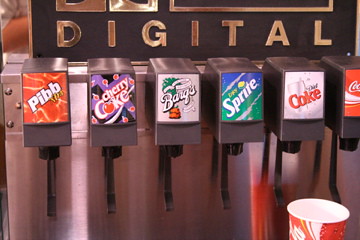The image depicts a fountain drink dispensary, possibly located in a movie theater, adorned with the word "Digital" in gold letters across the top. Below this, the stacked logos appear for six different soda options, each color-coded with their familiar brand colors: Pibb (orange background), Cherry Coke (black and red), Barq's Root Beer (light brown with dark brown lettering), Sprite (green background), Diet Coke (light background), and Coca-Cola (red) from left to right. Each soda is dispensed through small black levers with circular nozzles in front. A red Coca-Cola paper cup with white interior and design is positioned towards the bottom right, strategically placed beneath the Diet Coke label, resting on the presumed metal grate surface of the machine. The overall machine is silver-toned, sleekly aligned, and captures a familiar scene of beverage selection for the viewer.